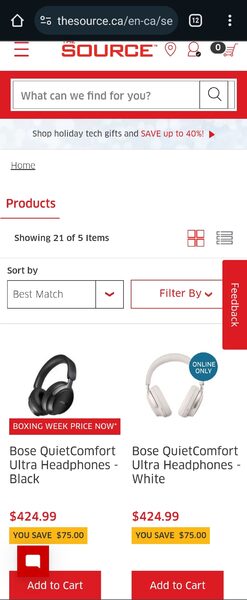This screenshot captures a segment of the webpage from "thesource.ca/en-ca/se." At the very top, encased in a black banner, is a search bar displaying the URL path. Beneath this bar, the brand name "The Source" is featured prominently in bold red lettering.

Directly below, within a red rectangle, is a white search bar posing the question, "What can we find for you?" This is followed by an advertisement encouraging shoppers to "Shop holiday tech gifts and save up to 40%."

The page indicates it is showing 21 out of 5 items, with options to "Sort by Best Match" and "Filter By" present. On the left side, there is a vertical red rectangle labeled "Feedback."

In the product display section, two pairs of Bose QuietComfort Ultra Headphones are showcased. On the left is a black pair marked with a "Boxing Week Price" tag, priced at $424.99, with a savings of $75. A blue "Add to Cart" button is directly below.

To the right, a pair of white headphones is depicted with a blue circle labeled "Online Only." These headphones carry the same price of $424.99 and offer the same $75 savings, accompanied by an "Add to Cart" button.

The screenshot is devoid of any human or animal presence, focusing solely on the products and web elements described.